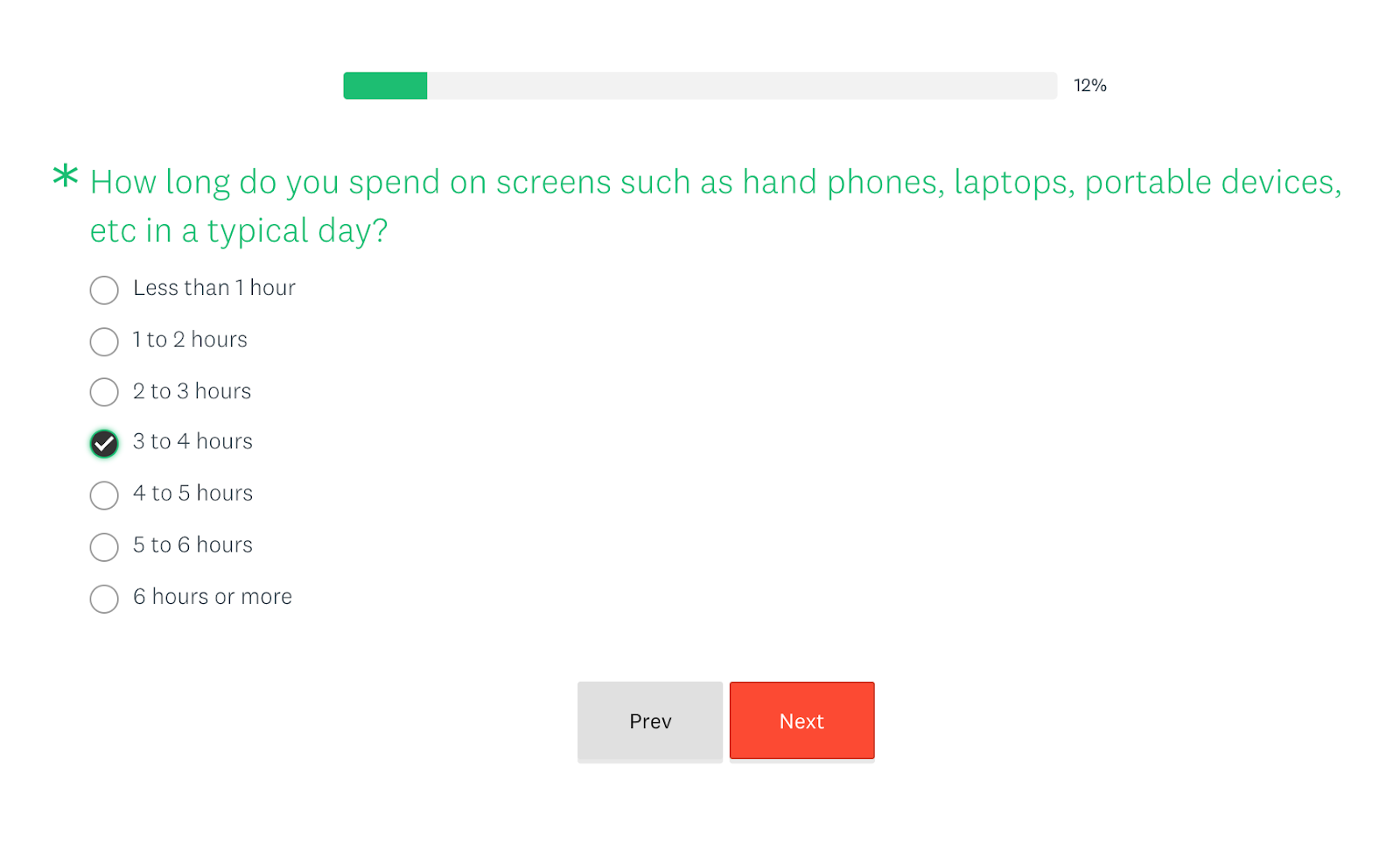The image features a survey question on a white background, without any borders. At the very top, a long horizontal ribbon is divided into two sections: a small portion on the far left colored dark green, and the rest in light gray. On the far right of the ribbon, bold black text displays "12%".

Below this ribbon, bold green text with a green asterisk at the beginning poses the question: "How long do you spend on screens such as handphones, laptops, portable devices, etc. in a typical day?" Underneath this question, a vertical list of options is displayed in black text, each accompanied by a white circle for selection. The options are:

- Less than one hour
- One to two hours
- Two to three hours
- Three to four hours
- Four to five hours
- Five to six hours
- Six hours or more

The option "Three to four hours" has been selected. Its circle is filled in black with a white checkmark inside and a light blue border around it.

Beneath the list of options, there are two rectangular buttons side by side. The left button is gray and labeled "Prev" in black text. The right button is orange or red, labeled "Next" in white text.